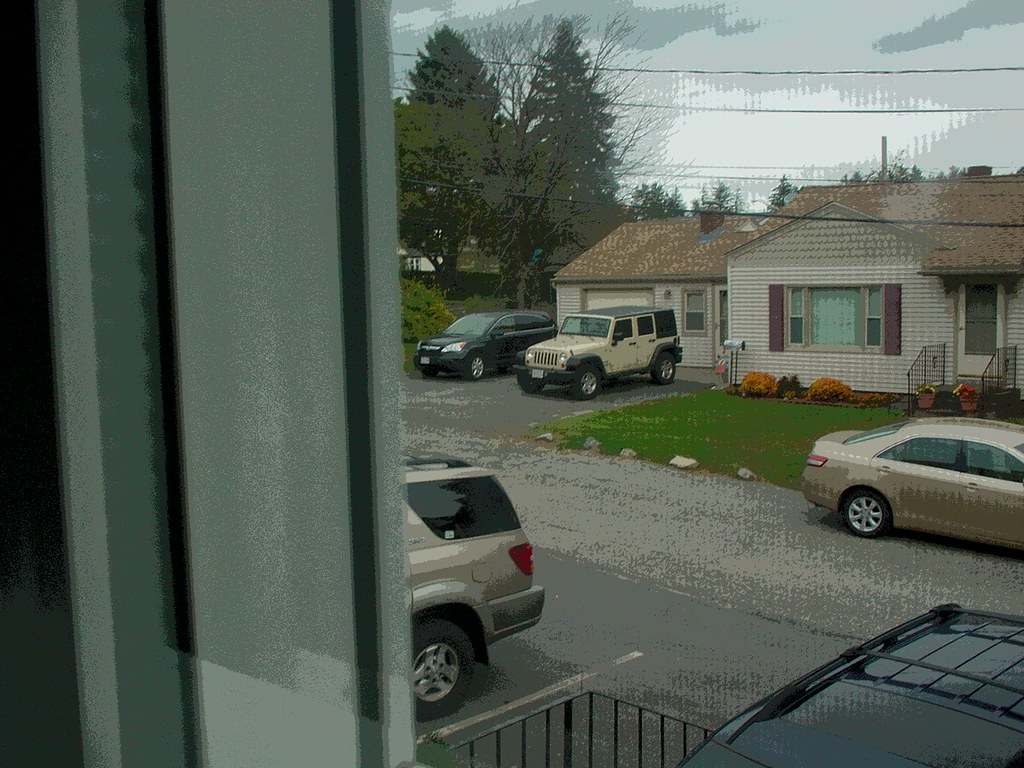In this horizontally elongated, vintage or lower resolution photograph, we are looking out through a window from inside a home. Outside, there is a view of a poorly paved street and a house across the way. The lower right corner of the image reveals the roof of a black vehicle parked beneath the window. To the left, we can see the rear end of a gold SUV parked in the driveway. The narrow, diagonal street slices through the image from the lower right to the upper left, with a gold car driving east on it.

Directly across the street stands a beige aluminum-sided ranch-style home, distinguished by red shutters adorning a large bay window. Positioned in the driveway in front of the garage, which occupies the left side of the home, are a beige, jeep-like vehicle and a black minivan, both oriented towards the street. The sky overhead is gray, casting a muted light over the scene. Adding to the quaint suburban atmosphere, two large pine trees stand majestically to the left of the home across the street.